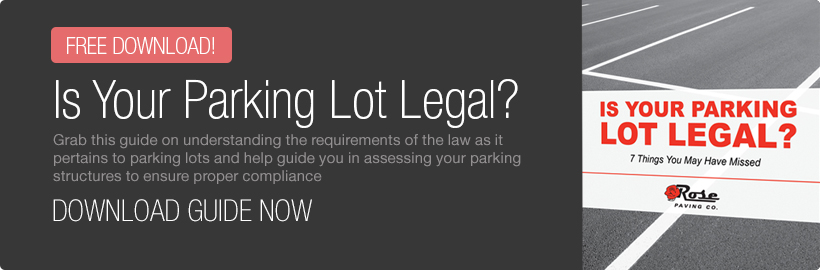This screenshot appears to be captured from a cell phone displaying a website for a downloadable app. On the left side of the image, there is a large horizontal black rectangle. In the top left corner of this rectangle, there is a smaller red rectangle with the text "Free Download!" in white font. Below this, in white text, it reads "Is Your Parking Lot Legal?". Further down in gray text, it provides additional information: "Grab this guide on understanding the requirements of the law as it pertains to parking lots and help guide you in assessing your parking structures to ensure proper compliance." Beneath this, there is a white text call-to-action: "Download Guide Now."

On the right side of the image, there is a vertical rectangle featuring a photograph of a paved parking lot marked with white lines delineating parking spaces. Overlaying the middle of this photo is a white banner with orange text stating "Is Your Parking Lot Legal?" and black text reading "7 Things You May Have Missed." Towards the bottom of this banner is an image of a red rose. To the right of the rose, in bold black cursive writing, is the word "Rose," and underneath it, in dark gray, lighter text, it says "Paving Company."